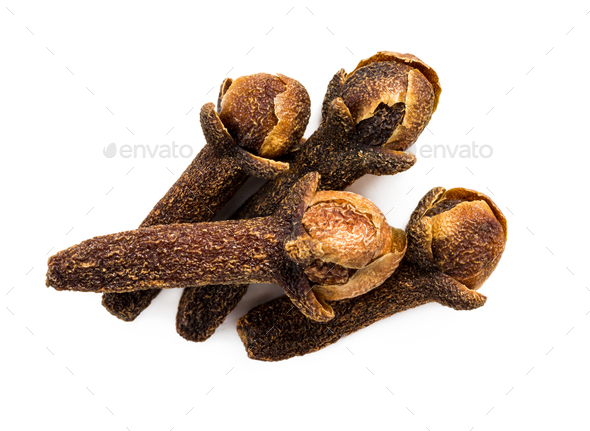The image shows a close-up color photograph of four cloves, a type of spice, set against a white background with faint cross-hatching and transparent gray text reading "Envato" on both sides, indicating it is a preview version of a stock image. The cloves are dark brown overall, with rounded tops in a lighter, golden-brown hue, some showing a peeling or shell-like texture. They have a cylindrical shape that flares outward at the top into an arch resembling flower petals, ending in a rounded head. Three of the cloves are arranged diagonally, appearing to fall from left to right, while the fourth clove lies horizontally across the others. The cloves feature a textured, speckled appearance, with narrowed, almost sharpened ends towards the bottom.